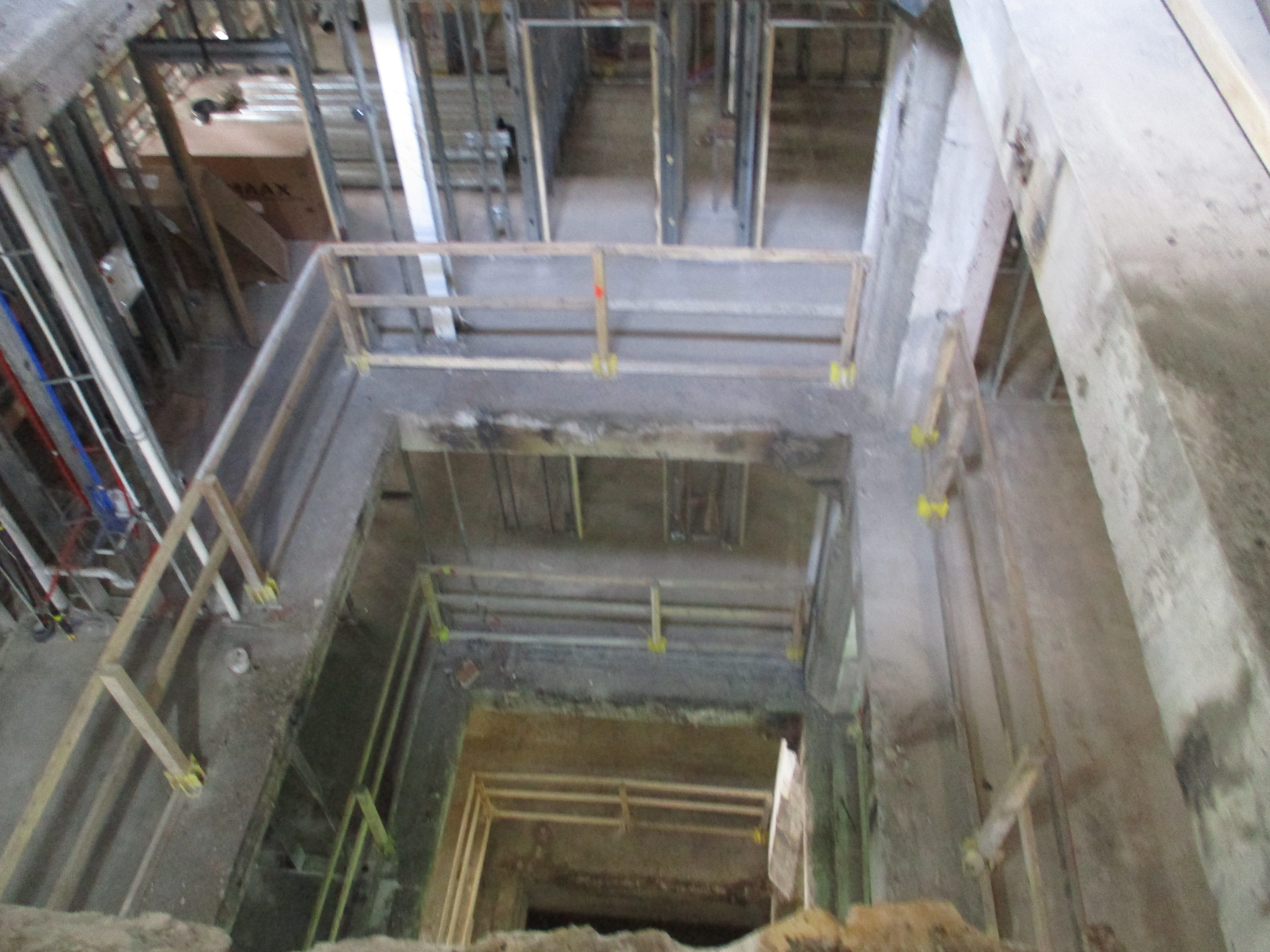The image depicts a multi-level structure under construction, featuring a series of concrete floors and exposed framework. The view is from the top level, looking down through a central opening that extends through at least five levels below, giving a sense of depth and unfinished potential. Each level has unpainted, light wood or white railings around the open center to prevent accidental falls, with yellow fixtures securing the posts. The exposed concrete walls and visible door frames hint at an incomplete state, possibly intended to become either an office building or a hotel. There are wooden boxes, perhaps containing supplies, on the left side of the top floor, and a ladder nearby, indicating ongoing construction work. The overall scene conveys a sense of raw, unrefined progress, emphasizing the skeletal stage of the building's development.